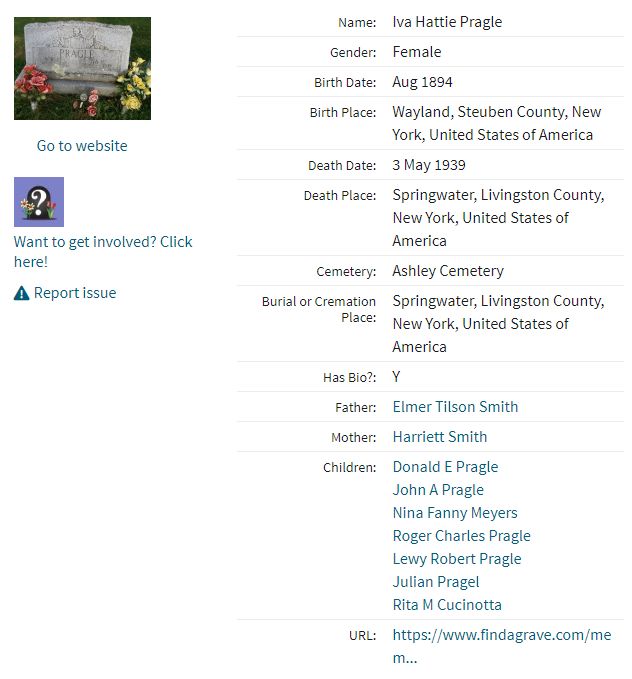The image shows a gray, rectangular stone grave adorned with pink and yellow flowers in front. The grave belongs to Ivor Hetty Prego, a female born in August 1894 in Wayland, Steuben County, New York. She passed away on May 3, 1939, in Springwater, Livingston County, New York, and is buried in Ashley Cemetery, also in Springwater. This information is presented as a snapshot from the website www.findagrave.com. The webpage features options such as "Go to website," "Want to get involved, click here," and "Report issue," with relevant links underneath. Additional details on the site include her name, gender, birth and death dates and places, along with fields to report issues or access further information.